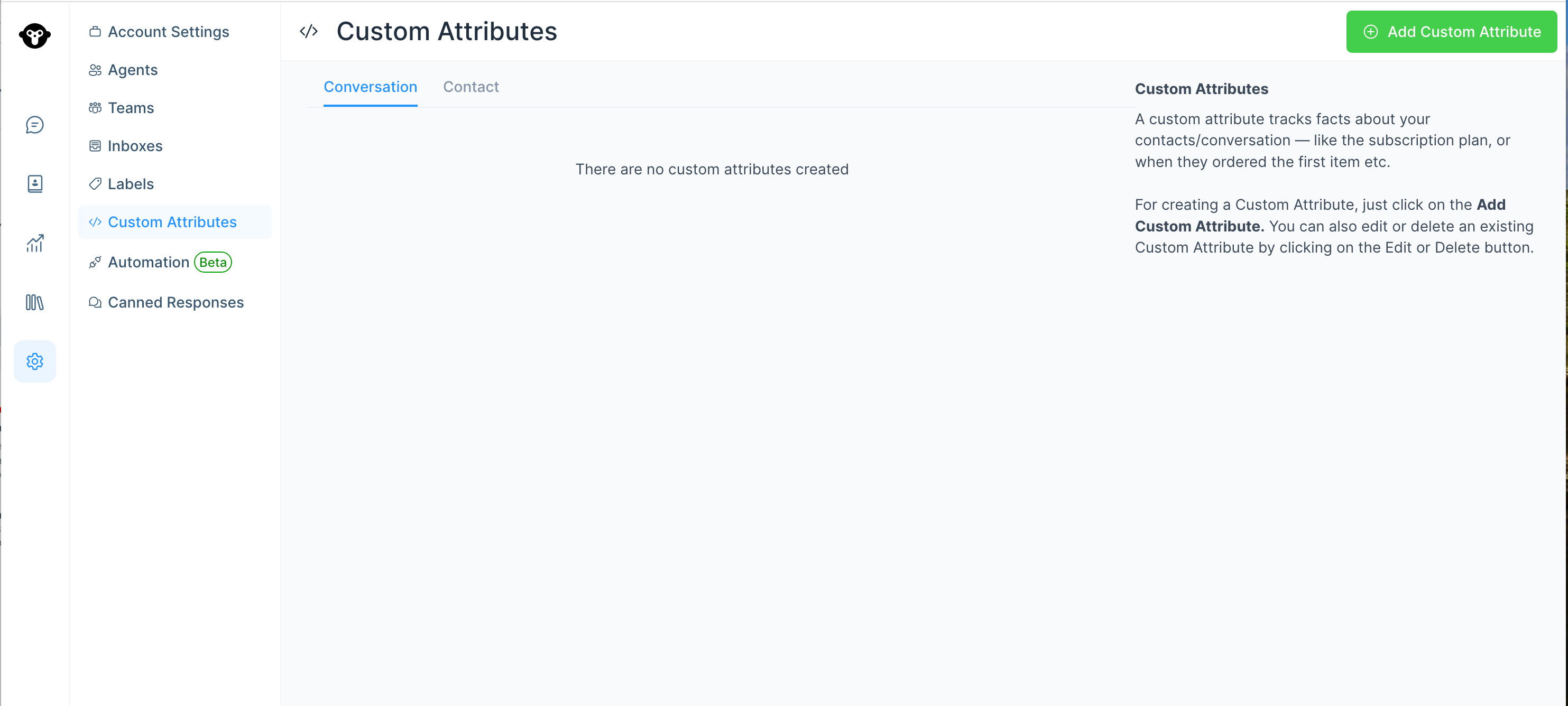The image captures a page titled "Account Settings" at the top. In the upper left-hand corner, there is an illustration of a monkey’s face. Moving downward, a vertical list of menu items appears, including "Agents," "Teams," "Inboxes," "Labels," "Custom Attributes," "Automation" (marked with a green oval labeled "Beta"), and "Canned Responses." On the left side of the page, there are various icons representing features, such as a speech bubble, a rectangle, stock charts, library books, and gears.

In the central section, under the header "Custom Attributes," there are subcategories for "Conversation" and "Contact," with a note indicating that no custom attributes have been created yet. On the right side of the page, a green button labeled "Add Custom Attribute" is prominently displayed. Below this button, there is explanatory text stating that a custom attribute tracks facts about the contact conversation, such as the subscription plan. Further information encourages the addition of custom attributes.